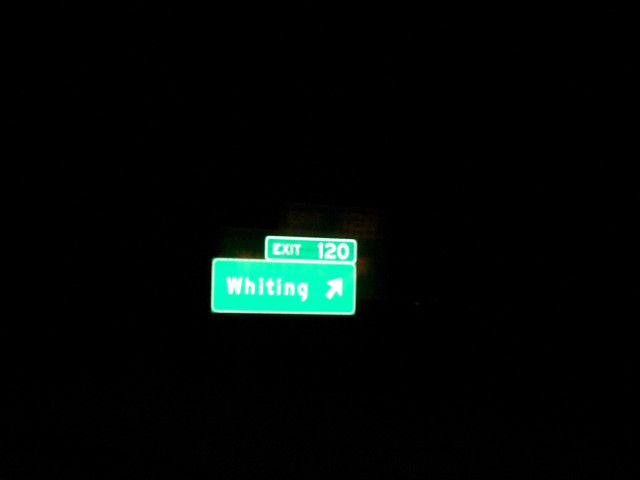This detailed, color photograph captures a pair of green traffic signs against a pitch-black background, making the signs appear as though they are floating in the darkness. The main sign, centrally positioned in the horizontal image, reads "Whiting" in bold white letters, with a thick, white arrow pointing diagonally to the upper right. Above this, another smaller rectangular green sign is attached, displaying "EXIT 120" in white, capital letters. The design and spacing of the signs suggest they urge drivers to prepare for an upcoming right exit toward Whiting. The absence of visible signposts or surrounding scenery indicates the photo was likely taken at night, emphasizing the stark contrast between the illuminated signs and the dark, empty background.